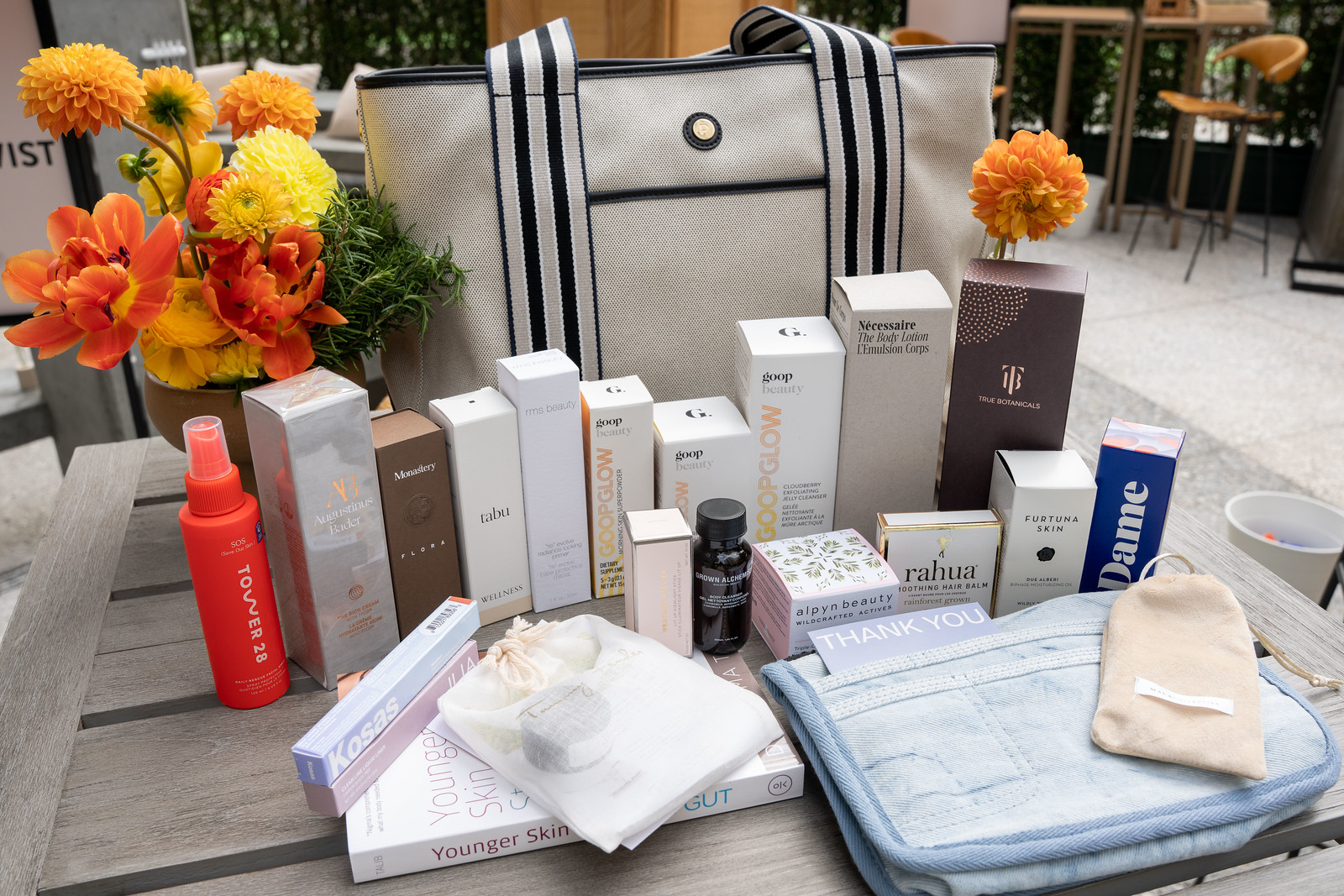On a table filled with an assortment of products, a grey bag with black and grey stripes catches the eye. Bright and colorful orange and yellow flowers adorn the left side of the table, blooming from a rustic brown flower pot, with a few stray weeds mingling among the petals. Among the neatly arranged products, there are several square and rectangular boxes, adding a geometric harmony to the scene. A small black bottle intrigued by its mysterious label written in a different language, and a blue and white box labeled 'Dame' stand out. Additionally, a small gift cloth bag reveals a dark, circular item within it. Adding a touch of vibrance, a little red spray bottle completes the display. In the background, the faint silhouette of chairs, which almost resemble tables, subtly frames the composition.